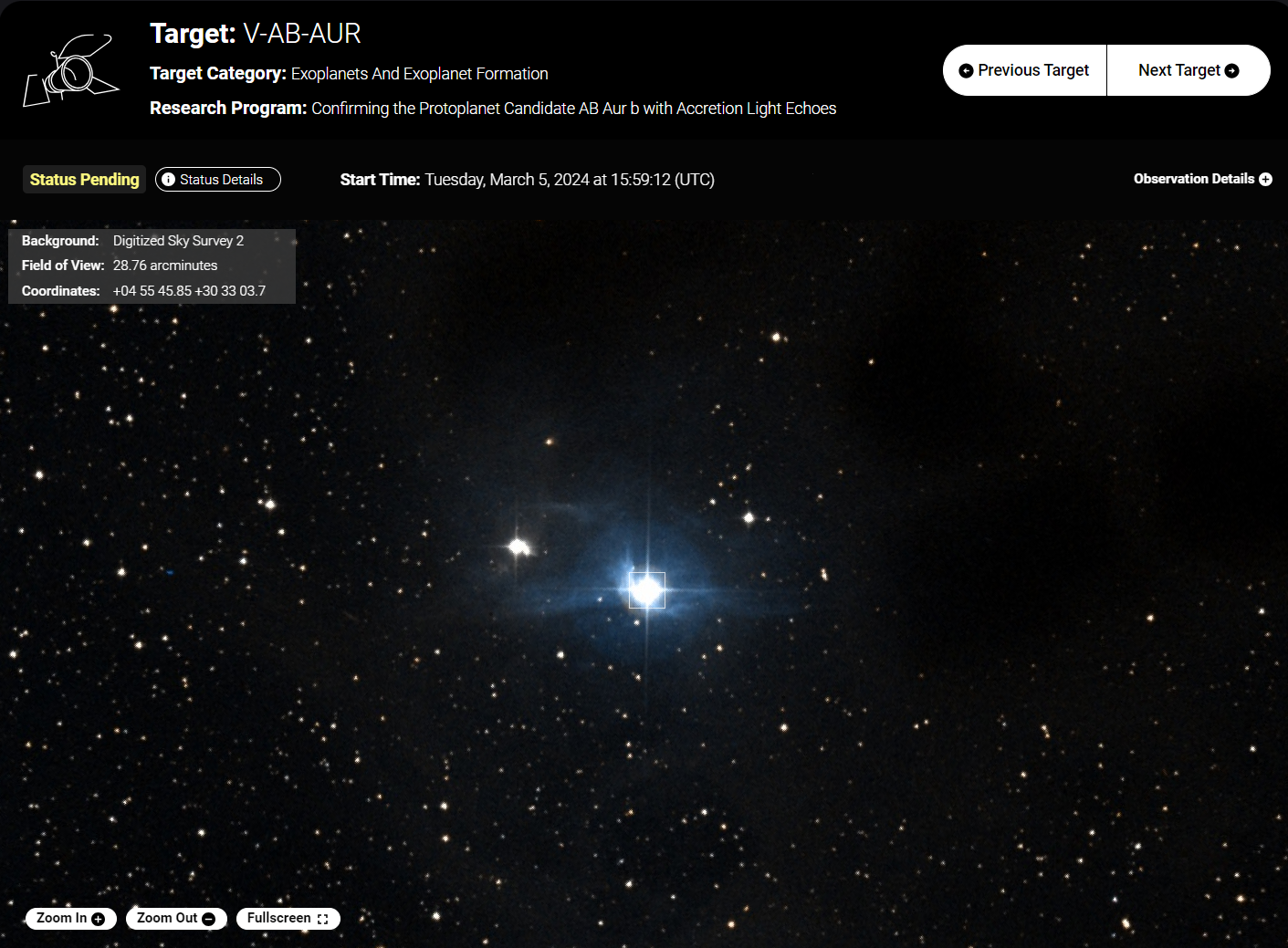This image is an astronomical program screenshot capturing a section of the night sky filled with stars, as observed through a high-powered telescope. The middle of the screen displays a black expanse punctuated by numerous stars, with two particularly bright, glowing objects that resemble headlights on a dark freeway, likely highlighting notable celestial bodies. In the upper left, a quadrant showcases a black border with white text that reads: “Target V-AB-AUR, Category: Exoplanets and Exoplanet Formation.” This section further mentions a "Research Program Confirming the Protoplanet Candidate" with "accretion light echoes," with a current "Status Pending." The top right corner includes navigation options labeled "Previous Target" and "Next Target" alongside a section titled "Observation Details." The start time for this observation is noted as Tuesday, March 5th, 2024, at 15:59 UTC. Additional information includes the background as "Digitized Sky Survey 2" with a field of view measurement and specific coordinates, though some details are not fully visible. The bottom left corner features zoom controls and a full-screen button, enhancing the interactiveness of this astronomical study tool. The image underscores the detailed efforts in confirming the existence of exoplanets through sophisticated observational technology.